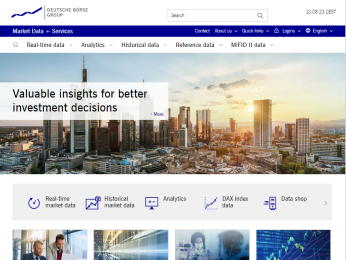The image depicts a webpage for a company or organization named "Deutsch [something] Group". The page's layout is as follows:

- At the top, there's a search bar positioned towards the right, next to some random text. 
- Below, a blue section contains navigation links including "Market Data and Services," "Contact," "About Us," and an option to switch to English.
- Another navigation bar below the blue section offers categories like "Real-Time Data Analytics," "Historical Data," "Reference Data," and "MiFID II Data."
- The hero section features a city skyline during sunset with a relatively clear sky and a few clouds. To the left of this image, there's a text section with a white background and black text reading "Valuable Insights for Better Investment Decisions."
- Following the hero section, there's a horizontally aligned section with five parts labelled "Real-Time Market Data," "Historical Market Data," "Analytics," "DAX Index Data," and "Data Shop."
- Lastly, there are four square pictures placed horizontally, each featuring various images with prominent blue elements.